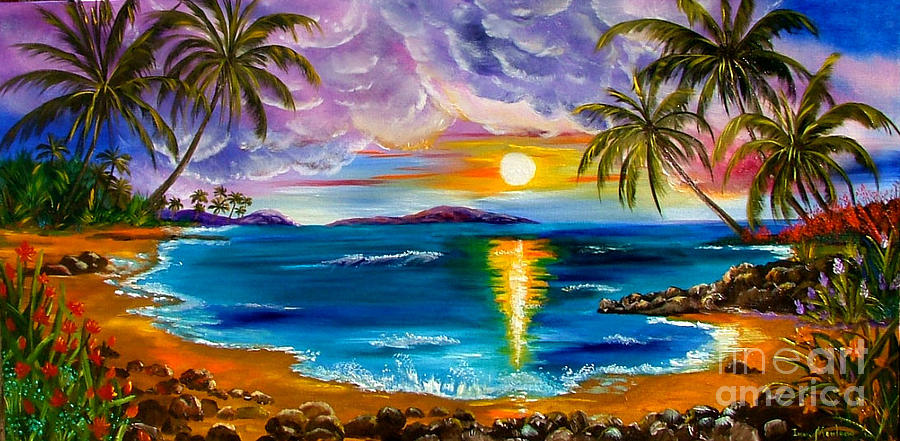The image is a detailed and vibrant painting of a tropical island beach at either dusk or dawn, featuring a breathtaking sunset. The sky is alive with purple, blue, pink, and white clouds, which almost appear translucent against the colorful background. In the middle of the sky, a bright, pale yellow sun casts long yellow and orange reflections across the ocean.

The U-shaped beach in the foreground is framed by dark brown sand speckled with round stones and rocks. The sandy shore is dotted with bright red flowers on the left and purple flowers on the right, adding a splash of color among the greenery. On either side of the cove, tall palm trees—two large ones on the left and three slightly smaller, bent ones on the right—lean gracefully over the water. Further in the distance, more palm trees and purplish mountains can be seen, enhancing the depth of the landscape.

The ocean itself is a mesmerizing blend of dark teal, blue, and even green hues, with white-capped waves scattered near the shore and towards the middle. The sun’s radiant yellow and orange streaks create a vivid reflection on the ocean's surface, melding beautifully with the water’s colors. White letters at the bottom right-hand corner of the painting indicate its origin, adding a subtle yet informative touch to this stunning portrayal of a serene tropical paradise.